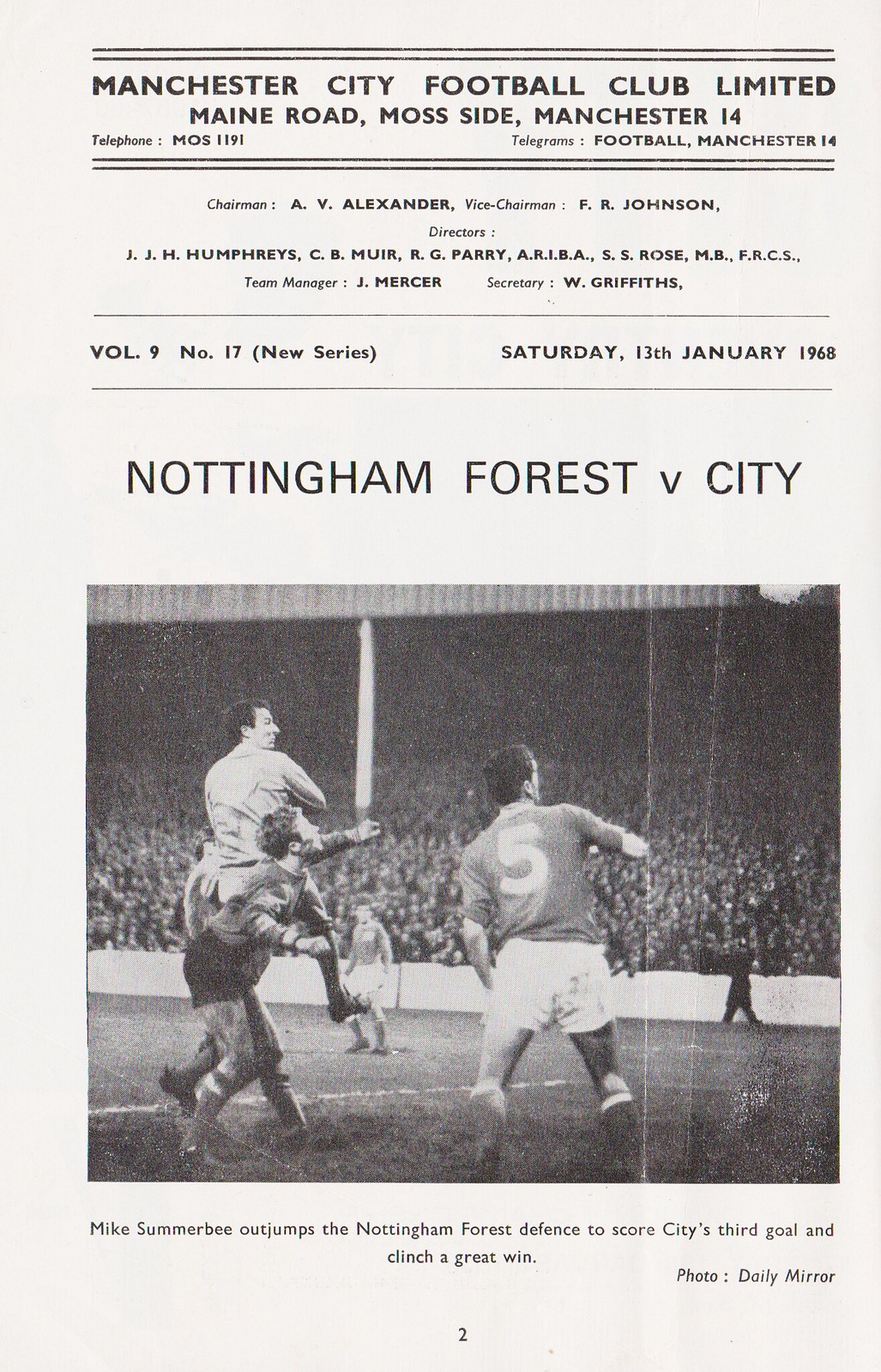A scanned magazine page in black and white, featuring a vintage print with a slightly off-white background due to age. The page is bordered at the top by double black lines and headline text that reads: "Manchester City Football Club Limited, Main Road, Moss Side, Manchester 14, telephone MOS 1191, telegrams: football Manchester 14." Below this header, an array of names and titles is listed: Chairman AV Alexander, Vice-chairman FR Johnson, Directors JJH Humphreys, CB Muir, RG Perry ARIBA, SS Rose MB FRCS, Team Manager Jay Mercer, and Secretary W Griffiths. This detailed header is followed by publication information indicating Volume 9, Number 17, part of a new series issued on Saturday, January 13, 1968. The match prominently featured is "Nottingham Forest vs. City."

The focal point of the page is a black and white action photograph set in a football stadium with a sizable, partially covered crowd in the background. The image captures several players in short-sleeved shirts and shorts, all looking up and to the right. Central to the image is a player with the number five on his back, seemingly outjumping others. To the left, two players appear to be colliding. 

The caption below the photograph reads: "Mike Summerbee out jumps the Nottingham Forest defense to score City’s third goal and clinch a great win. Photo Daily Mirror." Positioned at the bottom right of the page, it confirms the photo's source, and a page number '2' is placed centrally at the bottom.